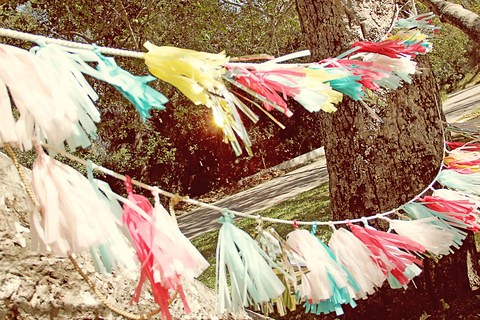The image depicts a horizontally aligned rectangular picture taken outdoors during daylight. At the forefront on the right side, there is a prominent tree with brown bark. Wrapped around the tree trunk are decorative strings adorned with colorful pom-poms or tassels, arranged in two distinct layers. The lower string features fringe in white, red, and blue, while the higher string exhibits similar decorations in a wider range of colors such as yellow, pink, blue, white, green, and red. The strings are tied securely around the tree and stretch toward another structure on the left side, forming a gentle curve.

On the left side, near the bottom corner, there is a large rock on the ground, surrounded by a patch of grass. The wind is gently blowing the tassels to the right, giving them a slightly elevated appearance. In the background, the image features numerous trees with lush green leaves, creating a dense backdrop that partially obscures the blue sky. The trees line both sides of a road that cuts through the middle of the scene, and sunlight filters through the foliage, casting light onto the road.